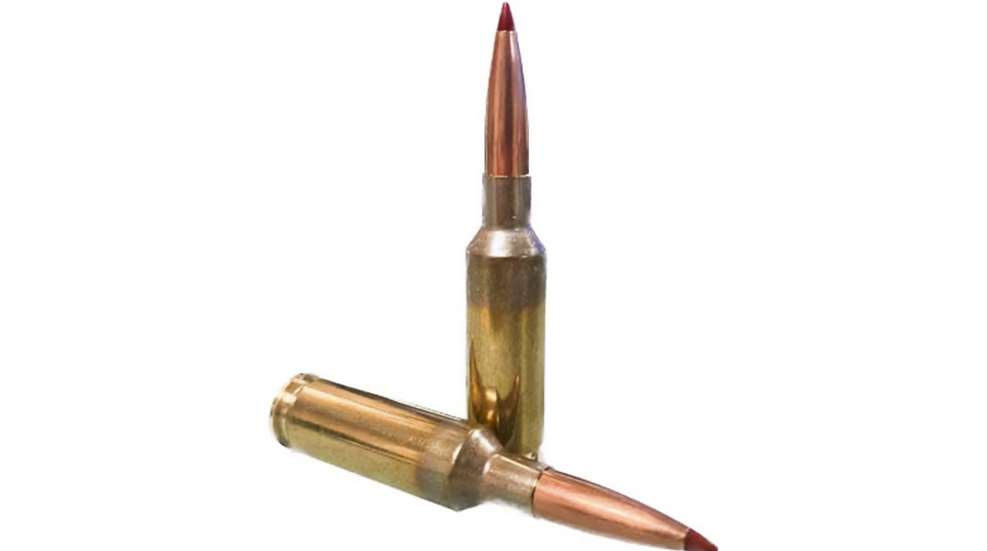The image features two large-caliber bullets set against a pristine white background. One bullet stands upright with a gleaming reflection at its base, reminiscent of a horned helmet, while the other lies horizontally next to it, oriented from top left to bottom right. Both bullets exhibit a gold-colored cylindrical casing that narrows into a brass-like projectile, which tapers to a pointed tip. The very tip of each bullet is distinguished by a dark reddish-brown color, deeper in hue than the coppery projectile beneath it. The overall design captures the intricate nuances of the bullets, from the brushed gold casings to the distinct coloration at their tips, possibly suggesting a product designed to resemble ammunition, though with a complexity that could also evoke comparisons to crayons or cosmetic items.